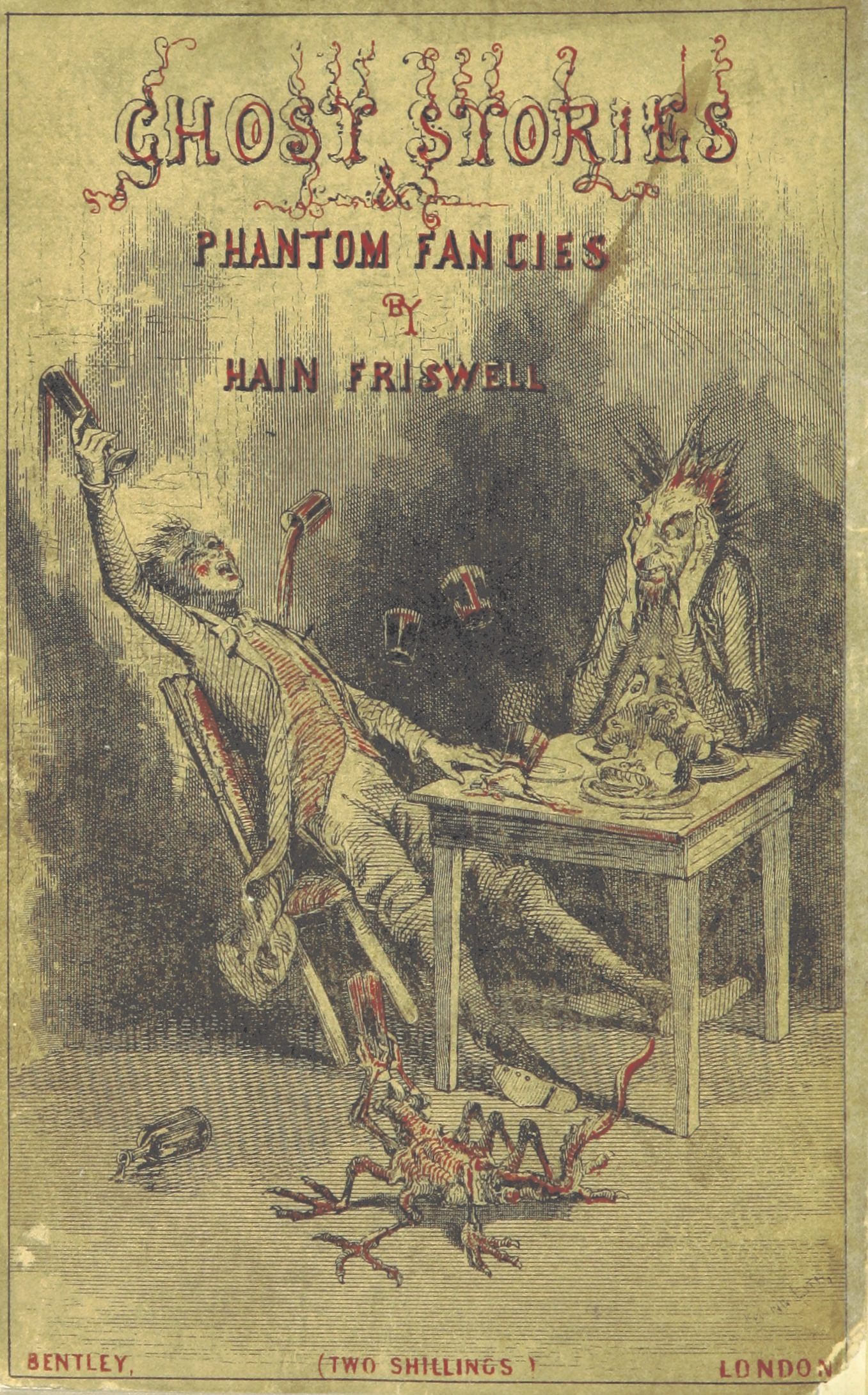This is the cover of a book called "Ghost Stories" with "Phantom Fantasies by Hayne Friswell" written underneath, both titles in a creepy red font with squiggly lines creating a shadow effect. The cover features a detailed sketch in shades of yellow, grey, and red. The scene depicts two monstrous figures seated at a table in a messy, dimly lit room. On the left, one character is a drunken young man, leaning perilously back in his chair while spilling liquid from a goblet. Multiple glasses are suspended in mid-air, one pouring a red liquid onto his chest. Across the table, a second figure with wild, spiky hair, wide eyes, and a beard rests his head in his hands, glaring at his unstable companion. The table is laden with a large roast or some kind of animal meat. At the bottom center of the image, a peculiar three-legged, scorpion-like creature is visible. The overall illustration is accented with splashes of red, including the text at the bottom of the cover, which reads "Bentley, Two Shillings, London." The book cover itself has a dingy, yellowish-olive hue, enhancing the eerie atmosphere.